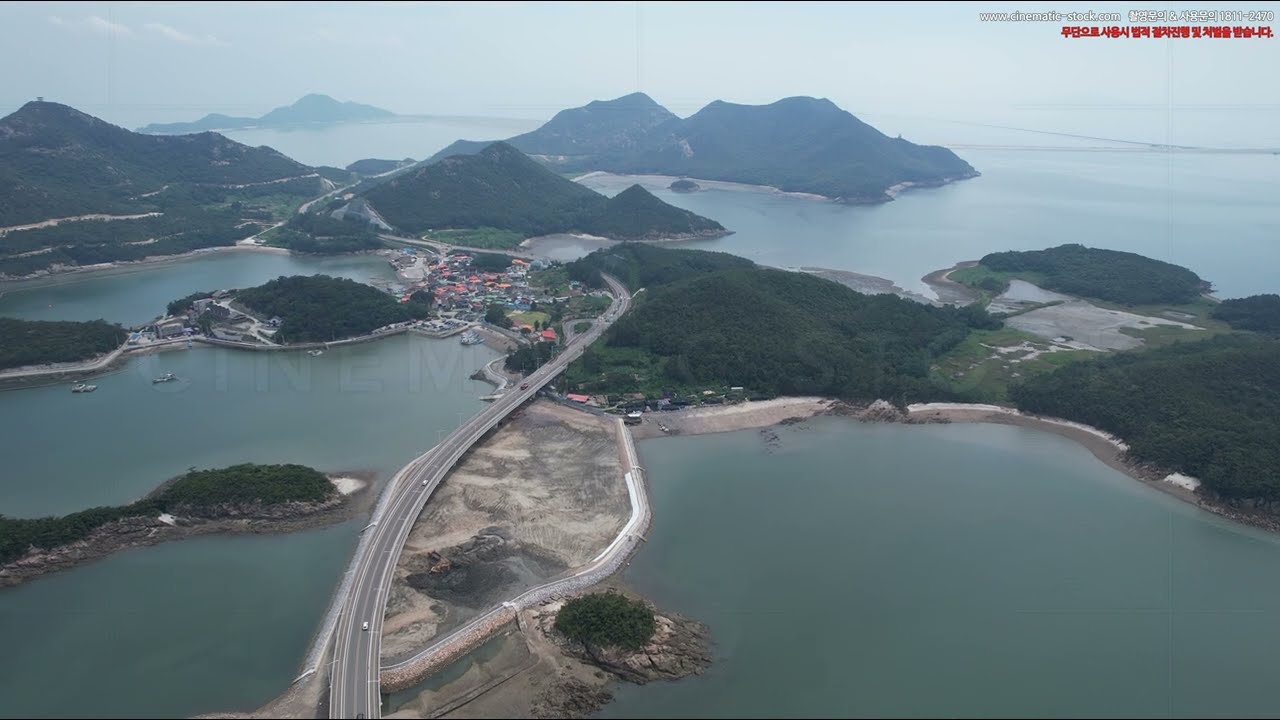A high-altitude daytime photograph reveals a scenic view of several small islands scattered throughout a greenish-blue ocean. Each island features lush green hills, with a particular emphasis on at least four larger islands near the top and two smaller ones on the left. A prominent curved road or bridge extends from the bottom of the image, weaving between the islands, and leading into a city characterized by numerous buildings with red or reddish-orange roofs. Towards the bottom, to the right of the road, a barren patch of land with a dirt-like appearance stands out. The image has an overcast sky, casting a grayish-blue hue over the scene. Additionally, there is a watermark in the upper right corner that reads "www.cinematic-stock.com" followed by Asian or Korean writing and the numbers 1811-2470. More Asian or Korean text in red is also present, indicating the photograph's stock origin.